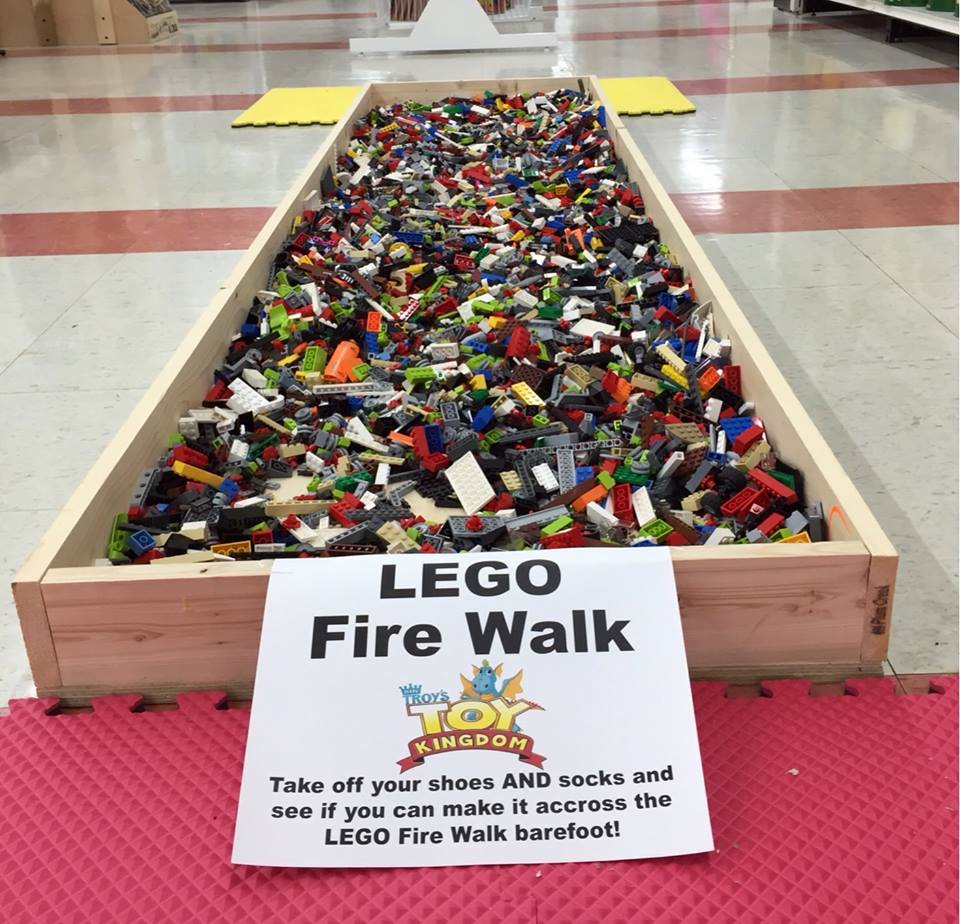In this image, we see a large, rectangular wooden container filled with colorful Lego pieces, positioned on a tiled floor—likely in a mall or school hallway. The container is approximately 10 feet long, 3 feet wide, and 4 inches deep, presenting a playful yet challenging obstacle. At the front of the container, a white sign prominently displays the phrase "Lego Firewalk," with a small emblem in the middle indicating sponsorship by "Roy's Toy Kingdom," featuring a dragon motif and vibrant blue, yellow, and red colors. Below this, the sign invites participants to "take off your shoes and socks and see if you can make it across the Lego Firewalk barefoot," daring onlookers to test their fortitude by walking over the notoriously uncomfortable Lego surface. The floor surrounding the display is tiled in white with red lines intersecting periodically, and the photograph zooms in closely on the container, capturing the essence of this engaging and whimsical challenge.